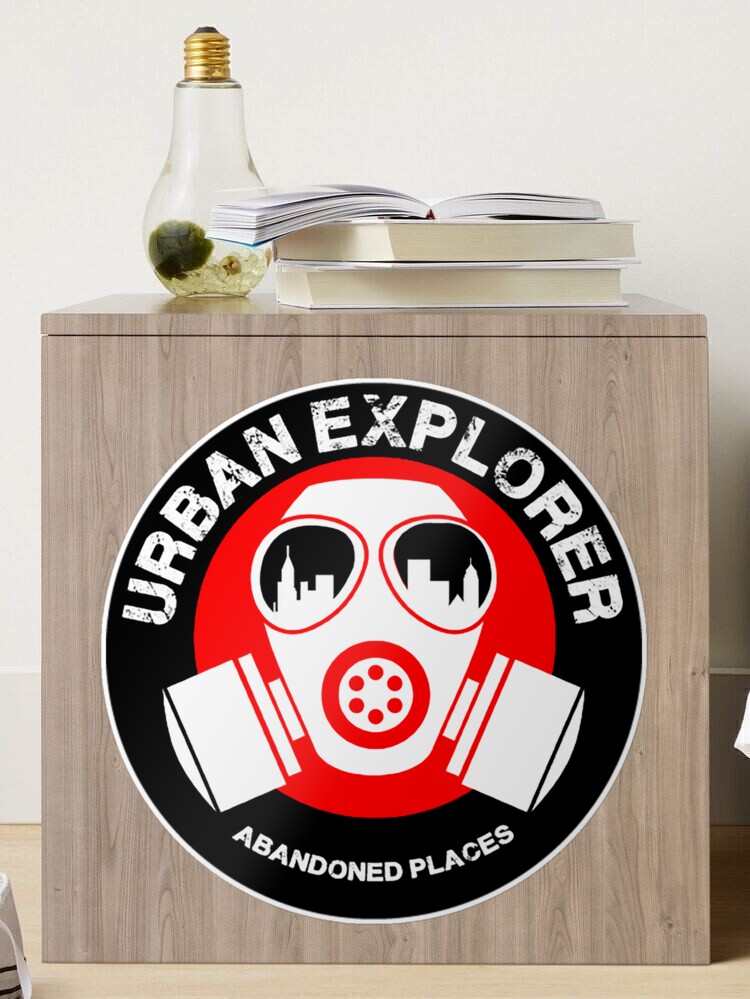The photograph captures the detailed scene of a small, rare-ish wooden table showing natural grayish patterns, situated in what seems like a lab. Centered prominently on the table's side is a distinctive circular sticker with a thin white outline and a black center, featuring a worn white text that reads "URBAN EXPLORER." Below this text, there's a striking emblem: a red circle showcasing a gas mask, with city skylines reflected in its goggles and a large red circle with small holes at the nose part. Adjacent to the gas mask design, the words "ABANDONED PLACES" are displayed. 

On top of the table, there are three books. Two of these are hardcovers, while the top one is an open trade book. To the left of these books, an inverted light bulb acts as a unique case, holding small objects that resemble rocks, almost giving the appearance of a miniature fish tank or terrarium with a moss ball inside. This carefully arranged tabletop scene is positioned against a wall, enhancing the photo's intricate and exploratory theme.